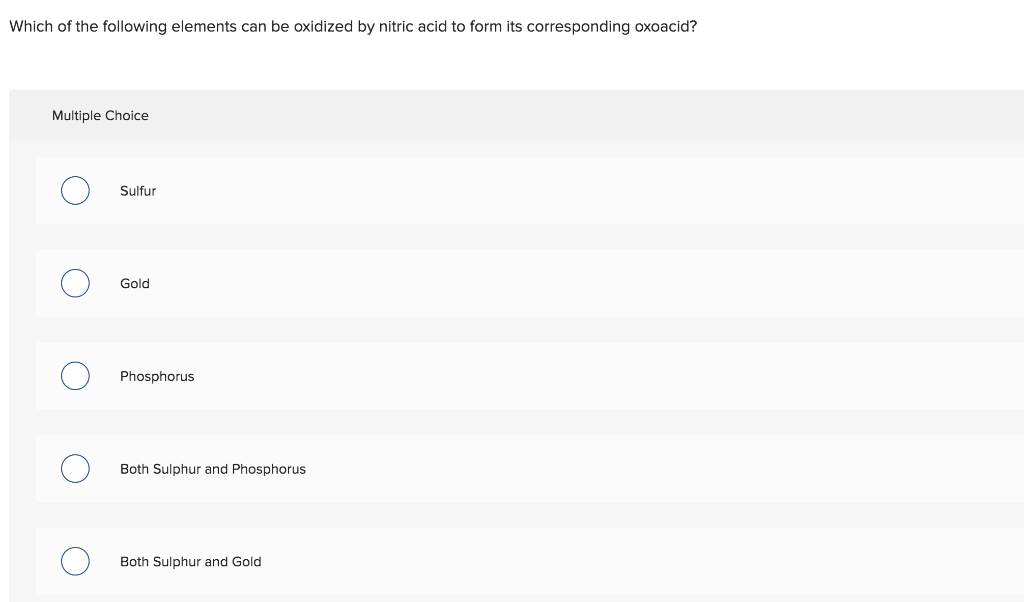This is a screenshot featuring a multiple-choice question from an unidentified source. The question at the top reads: "Which of the following elements can be oxidized by nitric acid to form its corresponding oxoacid?" Below the question, there are five options listed vertically, each accompanied by an unselected radio button. The choices are: 

1. Sulfur
2. Gold
3. Phosphorus
4. Both Sulfur and Phosphorus
5. Both Sulfur and Gold

The background of the screenshot is plain and contains no photographic or illustrative elements. Additionally, there are no people, animals, plants, buildings, flags, signs, vehicles such as motorcycles, automobiles, bicycles, helicopters, or airplanes, nor any depictions of water or food present in the image.